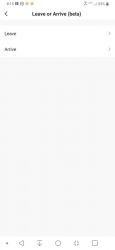This image portrays a very blurry smartphone screen, possible a selection screen, obscuring specific interface details such as battery level, Wi-Fi strength, and other top bar icons. At the top, just below a partially visible head bar, text reads "Leave or Arrive, Beta" accompanied by a back arrow, both of which are difficult to discern clearly. Below this are two large white overlay bars labeled "Leave" with a right-pointing arrow next to it, and "Arrive," separated by a thin gray line. Further down, occupying most of the screen beneath a significant gray space, sits a navigation bar. This bar features six distinct symbols arranged from left to right: a dot, a reverse arrow, a back arrow, a download button, a circle/play button, an asterisk, and a square positioned at the far right.